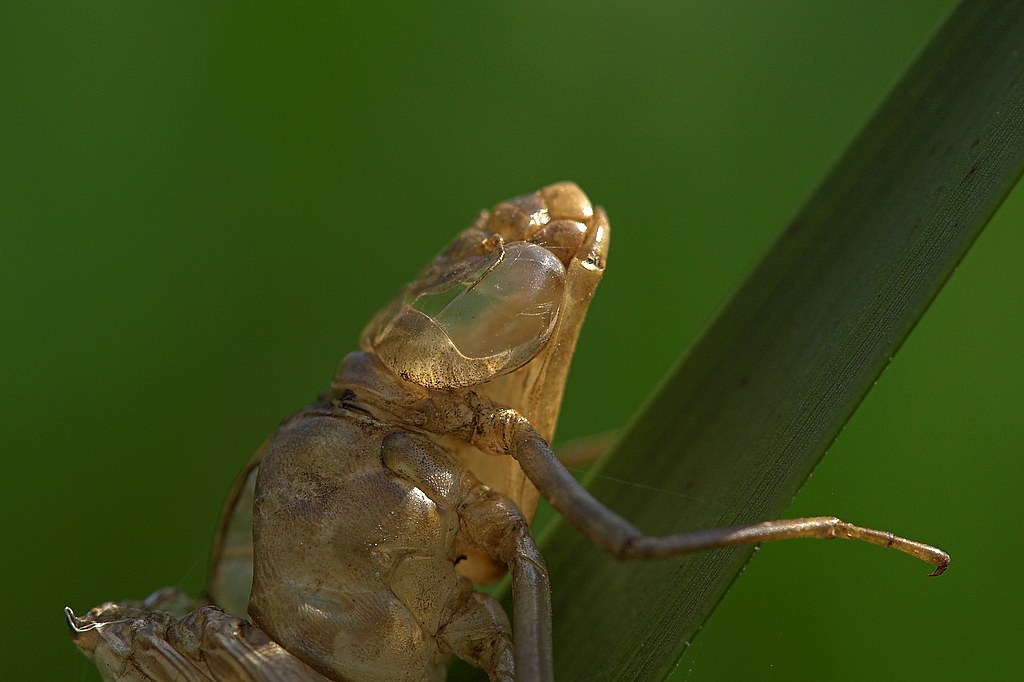This image captures a close-up view of a translucent, ruddy beige-colored insect, possibly the shed skin of a cicada or locust, perched on a thin, green blade of grass. The insect's head is partially out of the frame, and its body reveals detailed segmentation and striations, especially noticeable at the points where six legs are attached. Three legs are distinctly visible: one leg stretching fully forward, another partially visible and bent downward, and a third nestled near its body. The insect's back appears slightly clear with a brownish, hazy tint. The background is an unfocused, uniform green, providing a stark contrast that highlights the intricate details of the insect and the grass, reminiscent of an image you might find in a nature magazine or documentary.